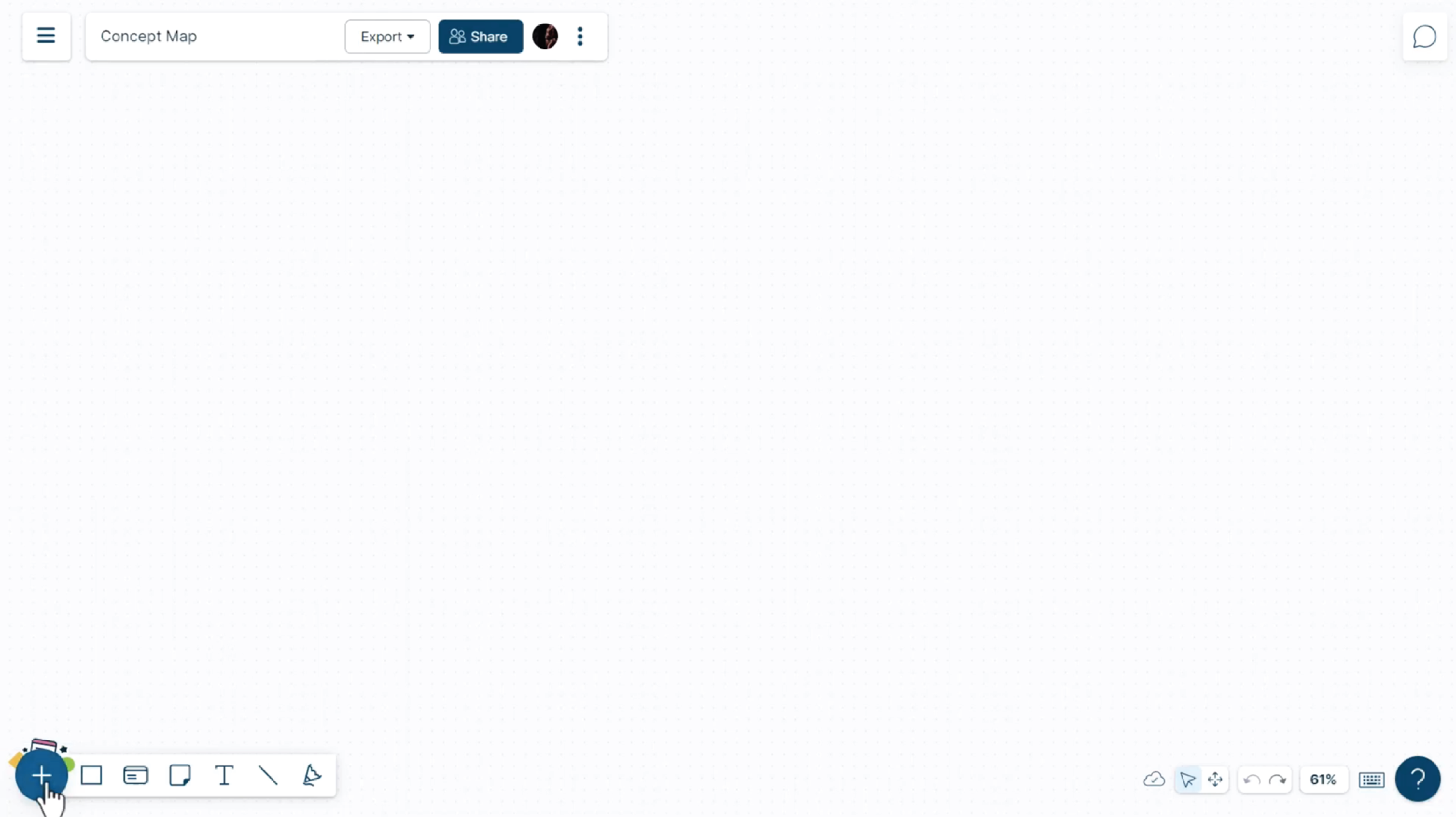**Detailed Screenshot Description:**

At the top of the webpage screenshot, there is a dark blue menu icon characterized by three horizontal lines. Below this is the address bar where a user would typically type in a web address or search query. This bar includes two tabs: the first tab labeled "Export" consists of a drop-down menu, while the second tab, designed in dark green with white letters, is labeled "Share." Adjacent to these tabs is a user profile icon followed by three vertical dots indicating more options.

The main body of the page is empty, presenting as a blank white background. Situated along the left-hand side of the page are various icons: 

1. A large greenish-teal circle with a white plus sign, pointed at by a hand icon.
2. A square box icon.
3. An icon resembling a file.
4. An icon of a piece of paper with a corner folded back.
5. A capital letter "T."
6. A backslash.
7. A pencil tip icon.

On the right-hand side, there is an icon depicting a cloud with arrows pointing in four different directions, signifying the forward and backward navigation functions contained within one button. 

Below this, there is a button displaying "61%," likely indicating a completion or progress status. Additional icons include a keyboard symbol and a help icon, which is a green circle featuring a white question mark.